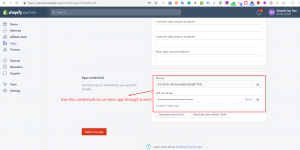A tiny, expanded image remains unreadable with text becoming illegible even when zoomed in. At the top, a light white bar extends horizontally from left to right, possibly indicating a browser window. On the far left, there are three distinct icons: a back arrow, a grayed-out forward arrow, and a refresh icon. To the right of these icons, an address bar is present. Following the address bar, 19 icons are lined up in sequence. Below this top bar, another horizontal bar spans from left to right. On the left-hand side of this lower bar, some white text can be seen, though it's unclear. To the right of the text, a search bar is evident. Further right, a notification bell icon is also visible.